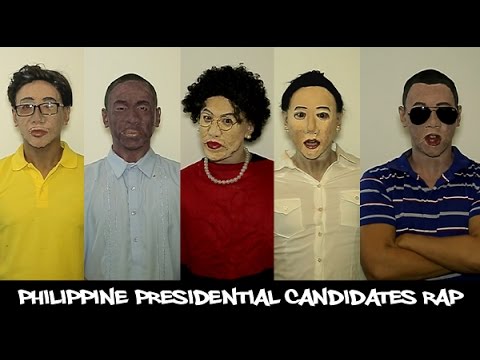The image features five people standing in a line against a predominantly white and light gray background, with thick black borders framing the top and bottom of the picture. The text at the bottom, in white graffiti-style capital letters, reads "PHILIPPINE PRESIDENTIAL CANDIDATES R.A.P." From left to right, we see: a man with brown hair and glasses wearing a short-sleeve yellow polo shirt; next to him, an African-descendant man in a long-sleeve blue dress shirt, with very short brown hair; in the center, a woman with short black curly hair, glasses, a red blouse, a white beaded necklace, and red lipstick; fourth is a person of unclear gender with short black hair, light skin, wearing a white button-up shirt with the collar open; and finally, a darker-skinned man with short black hair in a blue and white striped polo shirt and black aviator sunglasses, standing with his arms crossed. The image appears slightly computer-generated, especially in the facial expressions, and captures each person from the lower torso up.